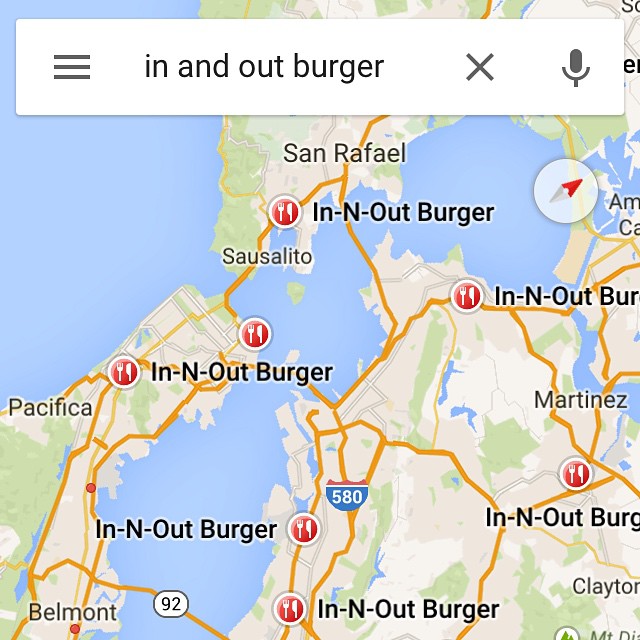The image is a detailed close-up of a map application showing search results for "In-N-Out Burger." The search bar prominently displays the query, and the map highlights multiple In-N-Out Burger locations. Key locations marked on the map include San Rafael, Sausalito, Pacifica, Belmont, Martinez, and Clayton, indicating a broad area of coverage mostly along the coast or near coastal regions. The map also features Interstate 580 running through its center, providing a sense of orientation. Additionally, the map showcases a body of water, likely the San Francisco Bay, and several green spaces that mark parks and nature preserves, contributing to the area's geographical context.